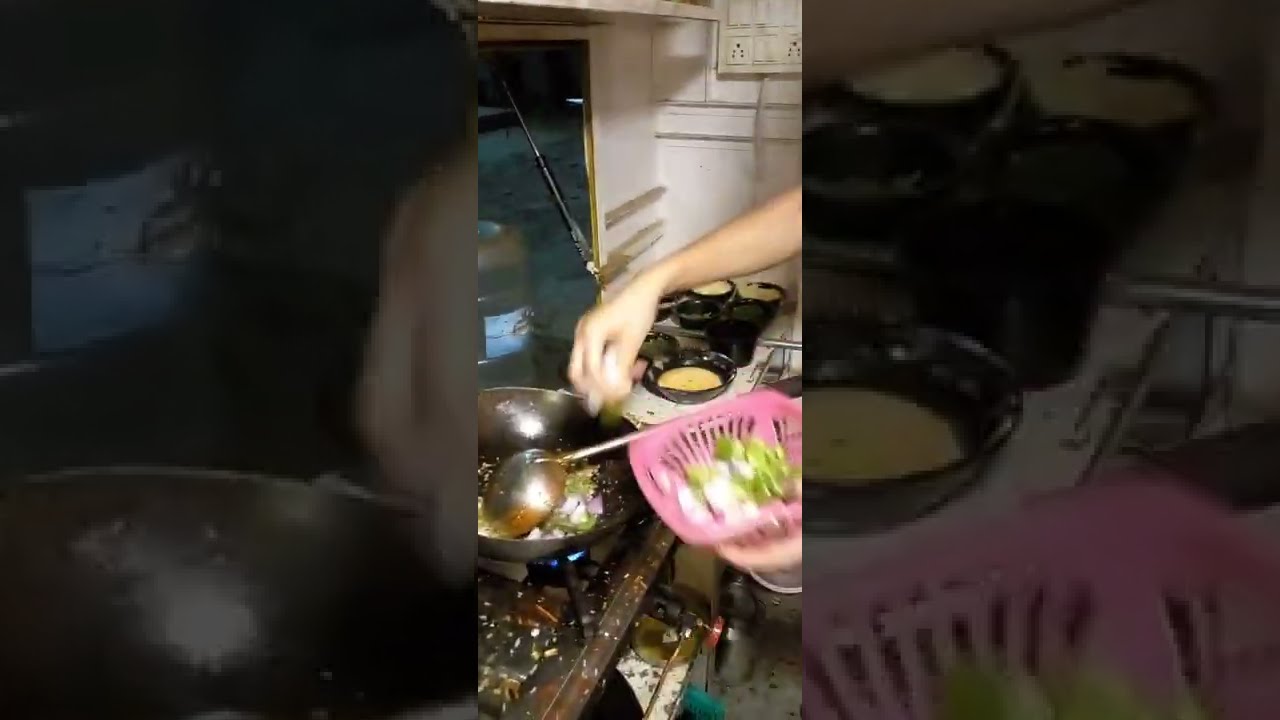The image is a vertical, cell phone-style photograph centered in a wider rectangular frame, which is notably wider than it is tall. The background on either side of the central panel is a zoomed-in and faded version of the same image, creating a cohesive yet blurred backdrop. The central image captures a cooking scene in a presumably messy kitchen with white walls. At the right side of the image, an extended arm appears, showing from just past the elbow to the wrist. The hand, which is blurry and appears in motion, is holding a pink colander or strainer containing a mix of white and green vegetables, likely onions and green peppers. The hand is dropping these vegetables into a black pan or small wok situated on a gas-powered stove, evidenced by the visible blue flame. Inside the pan, there is a chrome-colored ladle amidst the cooking vegetables. Additional details include several bowls with a saucy liquid positioned nearby. The overall scene suggests a dynamic moment of cooking amidst a cluttered kitchen setup.